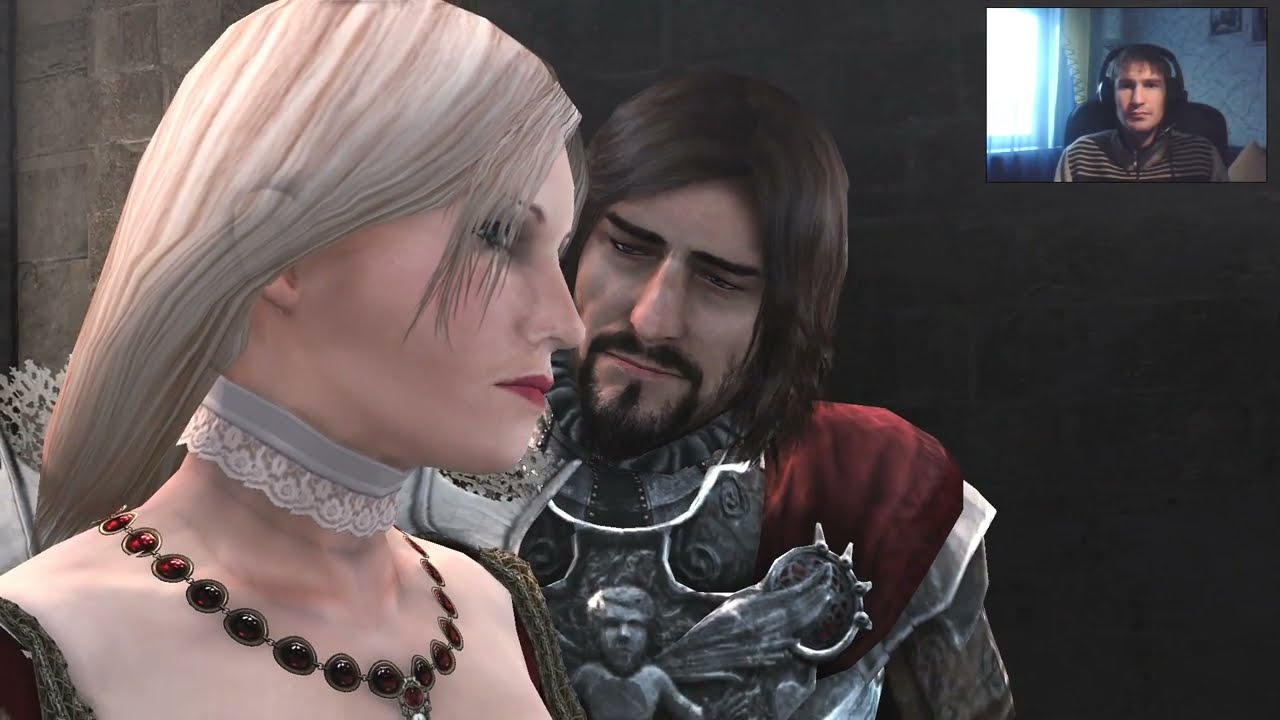This image is a detailed screenshot from a video game, featuring two characters in an intense conversation. In the center, a Caucasian woman with brown hair is visible, her mouth open in speech. She wears a low-cut ivory dress adorned with lace on the chest. To her left is another figure, partially visible from the back, dressed in a red and white, high-collared outfit reminiscent of royal attire. The background is dominated by a grey stone wall decorated with black metallic chains, giving a stark, medieval ambiance. In the top right corner of the image, there is a small rectangular inset showing a Caucasian male gamer with over-the-ear black headphones, sitting in a room with bright lights streaming through a window, and a black and grey striped shirt, presumably engaged in playing the game.